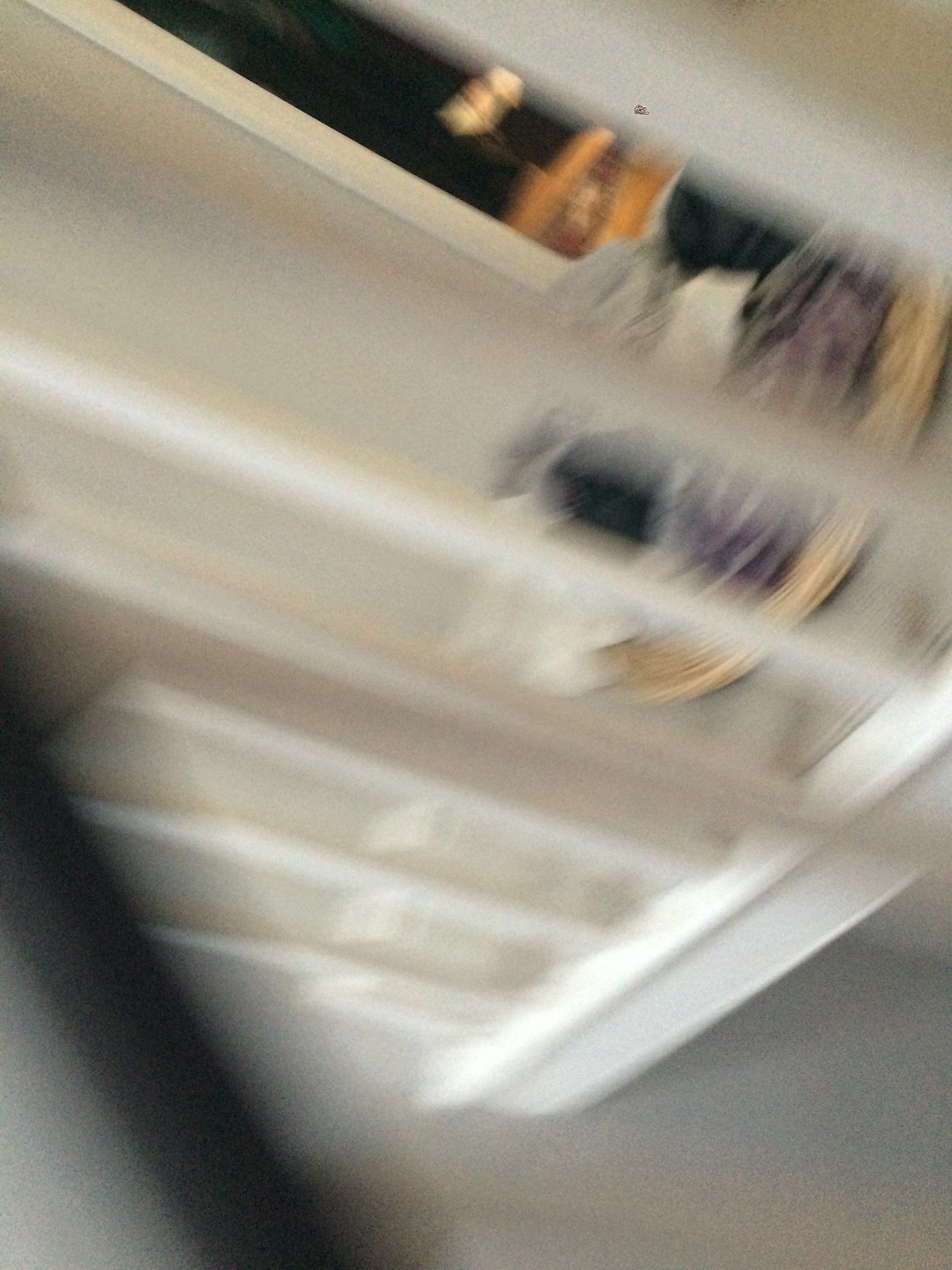A highly blurred image, challenging to discern. Prominent features include a black vertical stripe and a black diagonal stripe in the lower left-hand corner, contrasted by another black stripe in the upper right-hand corner positioned at a different angle. The indistinct suggestion of white shelves is also present, possibly indicating motion. Additionally, there is a white diagonal element intersecting in the opposite direction of the black stripes, creating a dynamic interplay of lines. The background appears to be gray, with a mix of eggplant-colored purple, tan, and orange hues in the upper right-hand corner. Overall, the image’s obscured and abstract nature leaves much to interpretation.